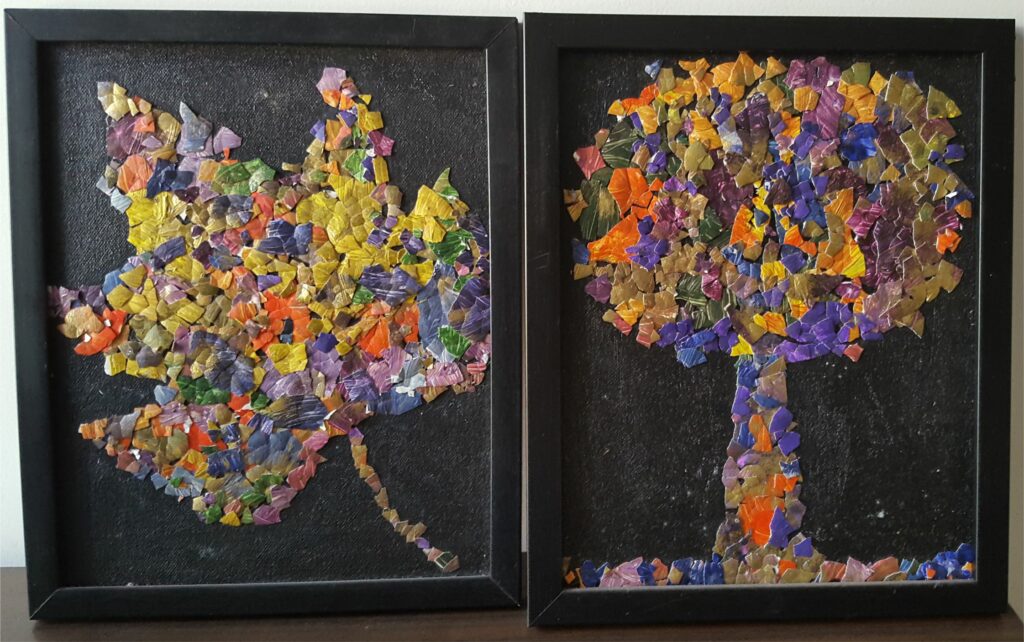The photograph showcases two vibrant pieces of artwork, both encased in sleek black rectangular frames against a chalkboard-like black background. The left frame contains an intricate collage forming the shape of a maple leaf, with its pointed tips oriented to the top left and a brownish stem anchoring it at the bottom. This leaf is composed of an array of vividly colored fragments, including shades of puce, turquoise blue, navy blue, purple, pink, orange, green, and more, creating a rich mosaic of colors.

To the right, in the corresponding black frame, is a similarly styled collage depicting a robust tree set upon a grounding surface. The elaborate tree is designed with a dense, colorful canopy filled with intense shades of orange, red, yellow, blue, and green, cascading down to form the grassy base. Both artworks, despite their different subjects, employ a consistent technique of fusing diverse colored materials—possibly crushed leaves, rocks, or paper—to craft their distinctive, eye-catching forms.